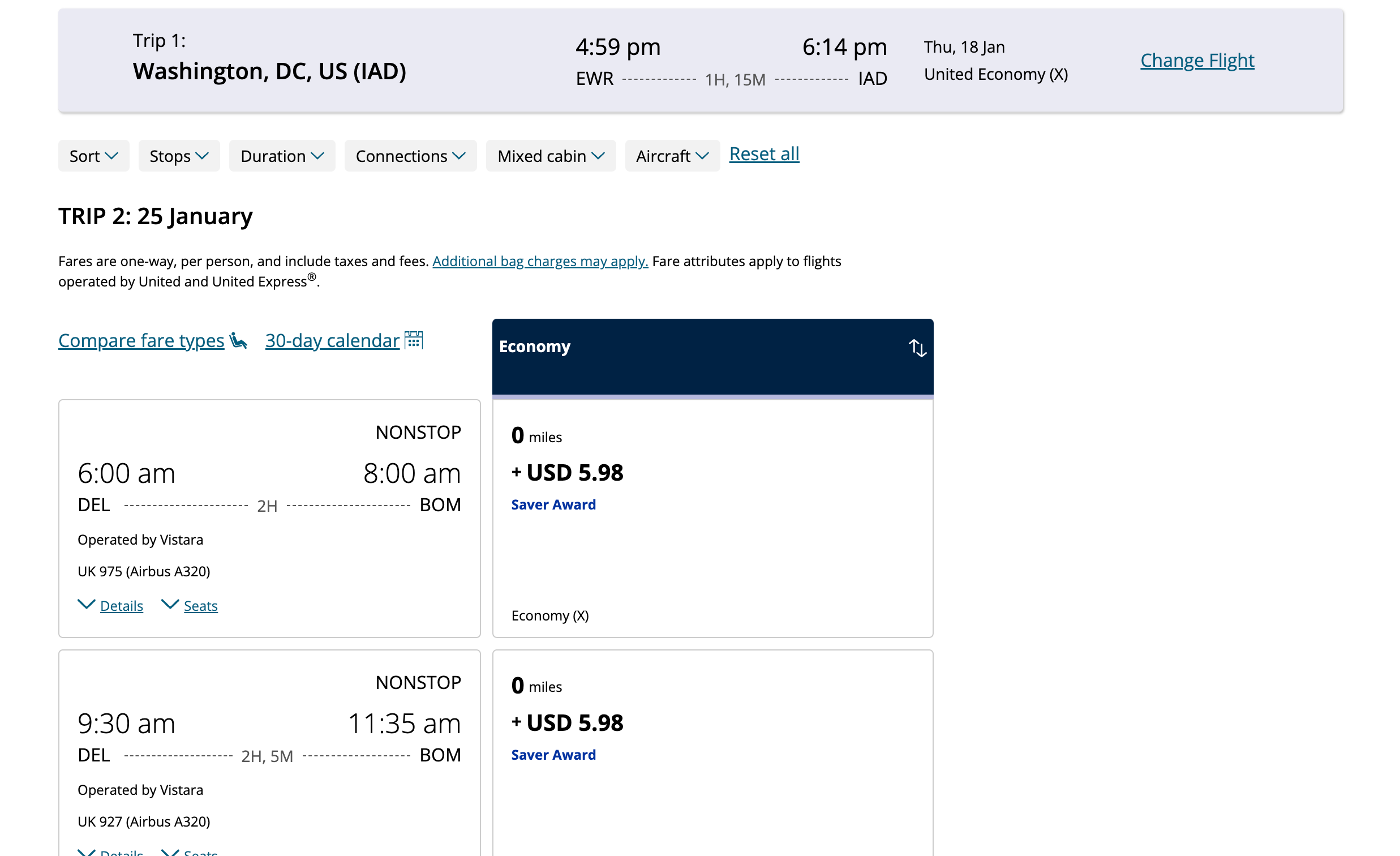The image features a top section with a gray border, containing travel details in various colors and formats. On the left-hand side, in black text, it reads "Trip 1: Washington, DC, US (IAD)." The middle part displays two time stamps: "4:59 PM" and "6:14 PM," followed by the text "EWR" (likely an airport code). Beneath the times, gray text states "1H 15M," indicating the flight duration. Further to the right, it says "THU 18 June" in black, with "United Economy (X)" written below. In blue, underlined text, there's an option to "Change Flight."

Below, a menu with tabs in gray and black displays options: "Sort, Stop, Duration, Connections, Mix Cabin, Aircraft." Additionally, a blue underlined option says "Reset All." Under this, it reads "Trip 2," in black text, followed by "25 January." A note mentions "Fares are one way, per person, and include taxes and fees," with an underlined blue text stating "Additional bag charges may apply." Another line in black specifies, "Fare attributes apply to flights operated by United and United Express."

Lastly, two sections list flight details: one section indicates a non-stop flight from "6 AM to 8 AM" and another from "9:30 AM to 11 AM," both marked as "Nonstop Economy." The first is priced at an additional "$598," while the second indicates "Zero miles Economy."